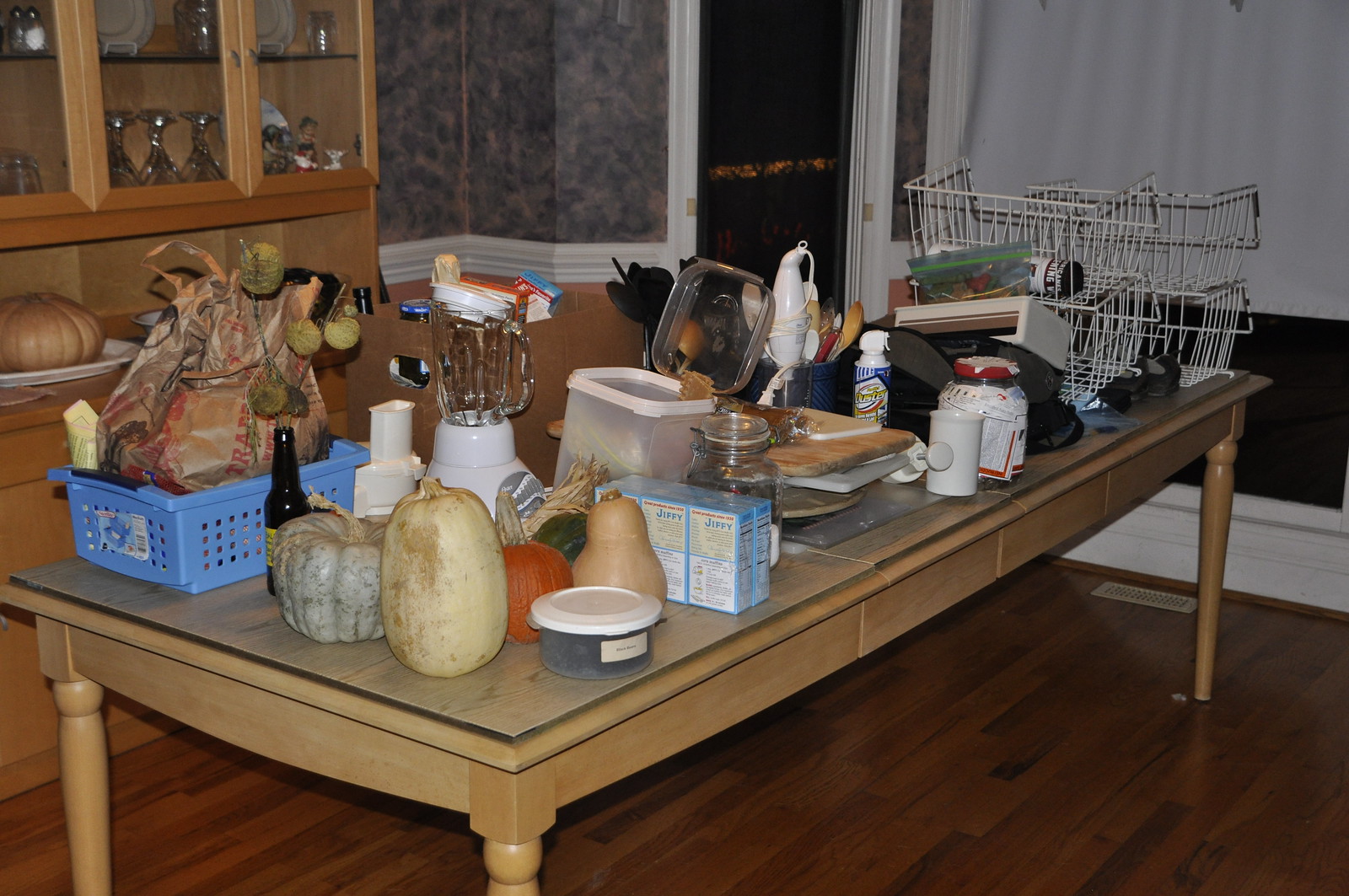In this photo of a cozy living room, a large light wood table occupies the centerpiece of the scene, adorned with a diverse array of items. Prominently displayed are artificial gourds and pumpkins, infusing a touch of autumnal charm. A vibrant blue basket holds a Trader Joe's bag, adding a burst of color amid the rustic decor. Nearby, part of a food processor and a blender sit ready for use, while several boxes of Jiffy corn mix await their turn in the kitchen. A glass mason jar and a plastic container with lids add to the eclectic collection on the table. Cutting boards and a bin filled with utensils lie alongside four white wire baskets neatly arranged at the table's end. In the backdrop, a large window with a drawn window shade allows natural light to filter in. To the left of the window, a doorway leads to another room, partially visible, with a glimpse of a partial wall. On the far left, a hutch filled with glassware completes the cozy, lived-in atmosphere of the room.